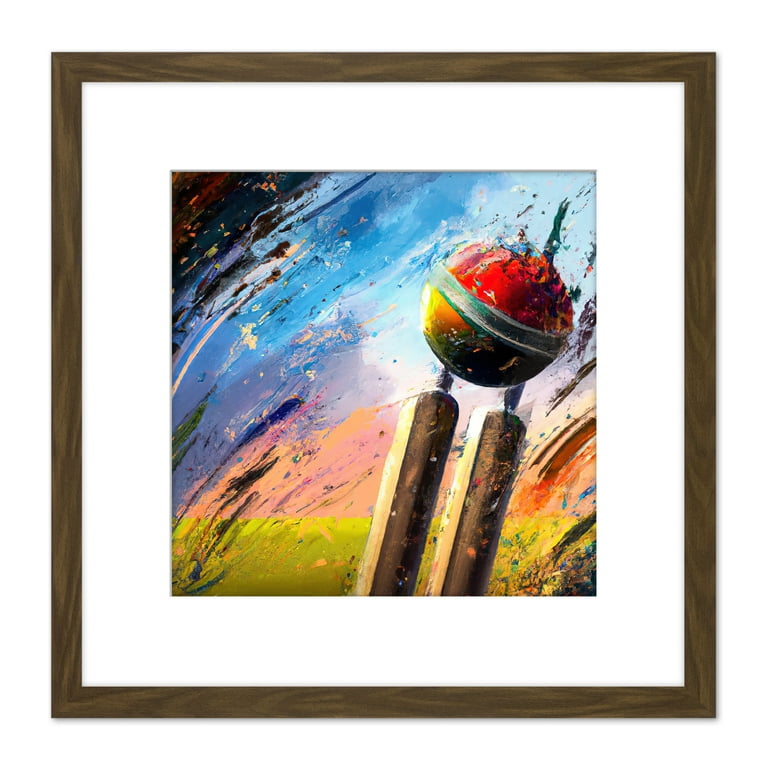The image is a vibrant, framed comic-book-style painting filled with an array of colors and dynamic elements. The wooden frame, digitally added with a dark wood effect, encases the painting with a thick white border. The centerpiece is a rich blend of muted yet bright hues: green reminiscent of grass, pink, lavender, yellow suggestive of a sunrise or sunset, with a gradient spectrum including purple, blue, and light blue leaning towards the right. Strewn throughout are black streaks that lend a menacing atmosphere to the scene. 

In the forefront, leaning towards the right and creating a sense of movement, two brown wooden legs or posts emerge, on top of which are metallic springs supporting a spherical object. This globe-like object is divided by a green seam running vertically, with its lower half glowing yellow and its upper half a deep red, symbolizing possibly a cricket ball or a Poké Ball. At the top of this sphere, a figure appears to be either breaking into or out of it. The painting includes a faint, barely legible signature in the bottom right corner, adding a touch of authenticity to this chaotic yet captivating artwork.